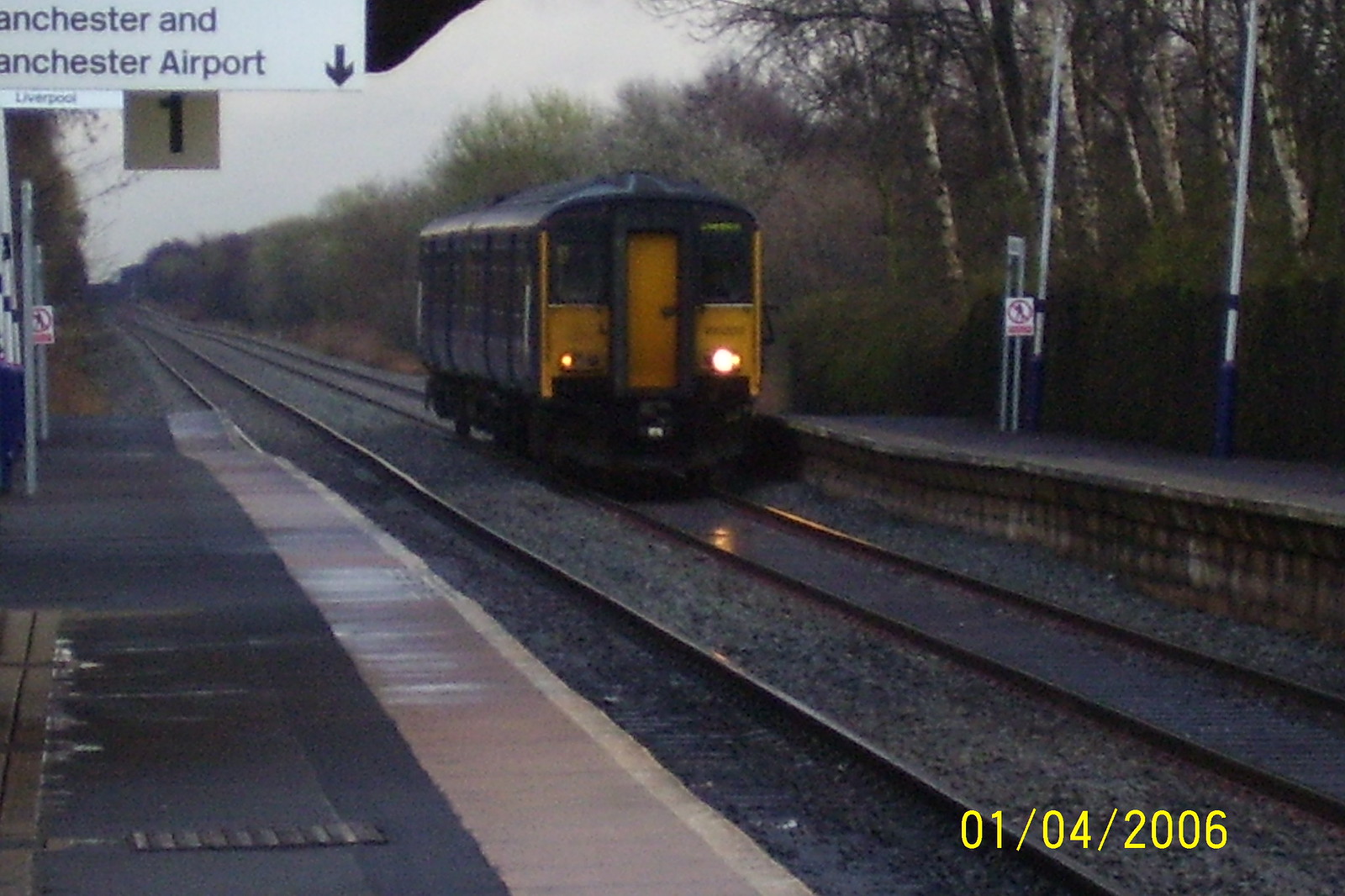A grainy, somewhat blurry photograph captures a lone yellow train car with a black top and illuminated front lights pulling into a station identified by signage as Manchester and Manchester Airport. The scene is set on a hazy, possibly foggy or smoky early morning or perhaps at dusk, under overcast skies. The train, appearing small and without passengers or waiting individuals, comes to a stop at Platform 1, indicated by a sign in the top left corner. The tracks, spanning from the bottom right corner of the image where a date stamp reads January 4, 2006, cut diagonally through the scene to the top left, surrounded by gravel and raised concrete platforms. On either side, lush green trees interspersed with red and yellow foliage frame the railway.